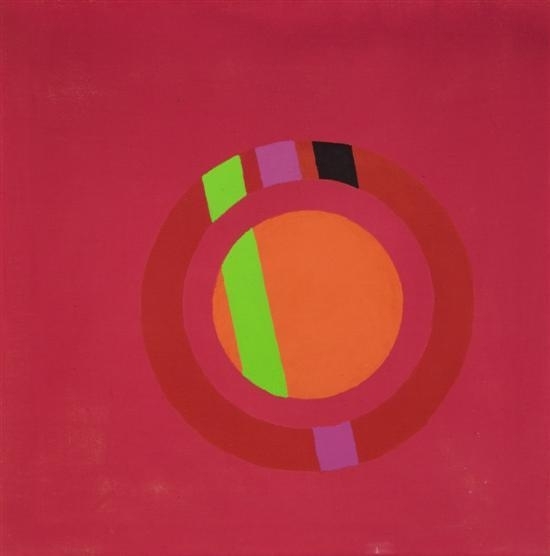Against a modern art painting's magenta-like, solid red background, lies a central composition of geometric shapes. Dominating the middle is a large, deep red circle with distinctive details. Cutting through this red circle is a vibrant, fluorescent green line that starts at the top, continues down the center, and fades as it approaches the bottom. The green line intersects an internal orange circle nestled within the red one. At the top section of the red circle, a streak of purple aligns directly with another purple streak at the bottom. Adjacent to these, a short black stripe is visible to the right of the top purple streak, while the light green line crosses over the orange center.

Encircling this structure is another outer ring in a pinkish-red hue, partially obscuring the inner circles and stripes. The overall precision of the artwork is highlighted by clean lines with minor jagged edges, adding a touch of meticulous detail. The background remains solid red, with subtle specks in the bottom left corner and faint brushstrokes of white paint, emphasizing the painting's textured and layered nature. This piece embodies modern use of shape and color, presenting an intricate interplay of circular patterns and ribbon-like lines.